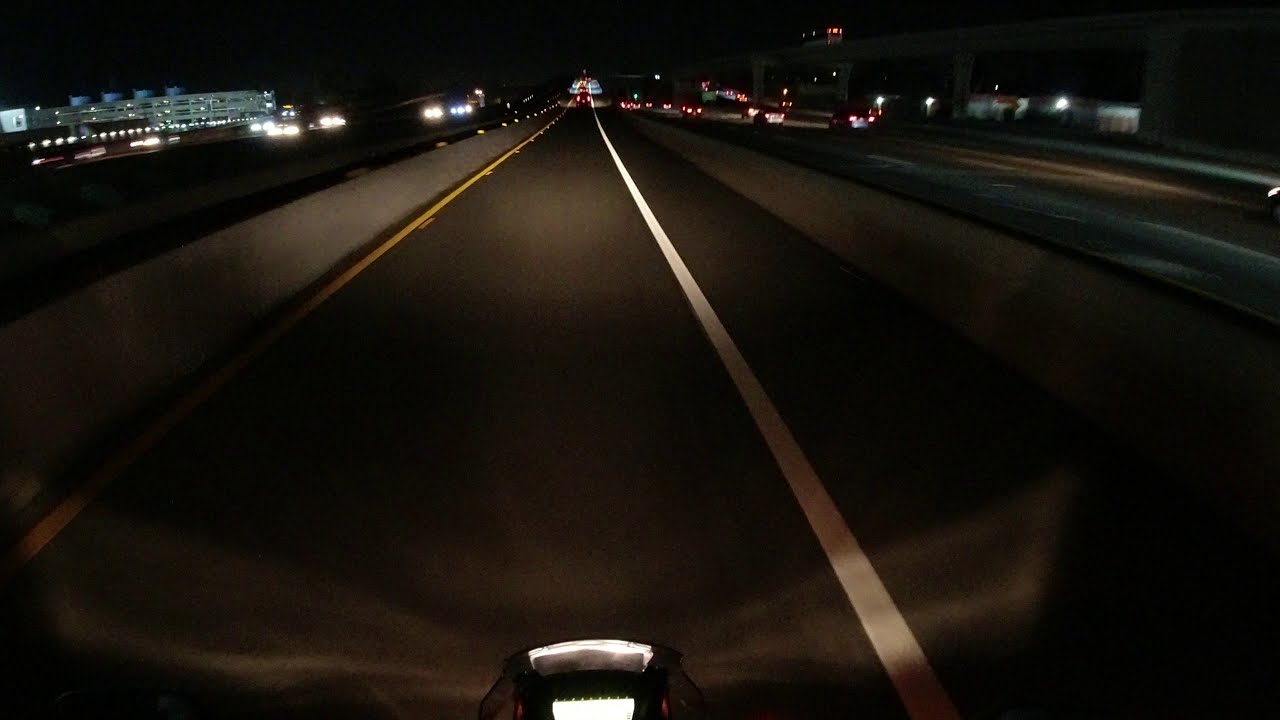The full-color nighttime photograph depicts a busy, multi-lane roadway with black asphalt, seen from the perspective of a motorcycle, evidenced by the prominent headlight at the bottom of the image. The road is framed by a solid white line on the right and a solid yellow line with dashes, running adjacent to a concrete barrier, on the left. This suggests the scene may not be in the United States. To the left of the barrier stands a gray, three-story building, illuminated but nondescript. The road is flanked by concrete barriers on both sides, beyond which lie additional lanes of traffic. On the right, vehicles are moving away, their red taillights receding into the distance. On the left, approaching vehicles display white, blue, and yellow headlights. Further along, in the dimly lit background, low-lying buildings, possibly corporate structures, are visible. The overall scene captures the bustling activity and layered structure of an urban roadway at night.